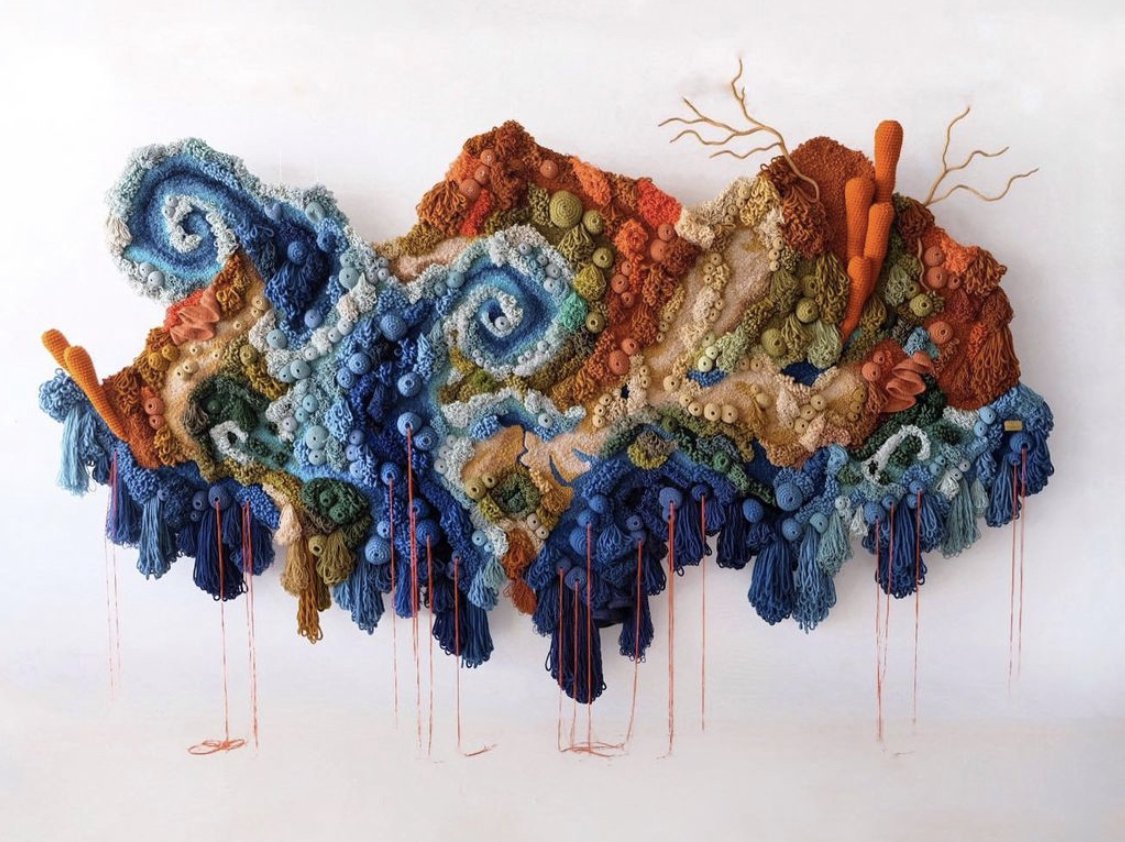A vibrant, abstract tapestry adorns a stark white wall, blending art and texture in an intriguing display. The fabric masterpiece features an array of colors including reds, blues, corals, burgundy, green, and white, creating a dynamic mural-like effect. Swirls of blue reminiscent of waves provide fluidity and mystery, while red, coral, and blue tassels with dangling, round elements add a three-dimensional quality. The intricate design includes fabric formations resembling bare trees, cacti, and colorful mountains. On the right side, orange carrot-shaped fabric pieces protrude amidst wavy brown tree branches, while the left side showcases an expansive blue spiral wave. The bottom of the tapestry is adorned with delicate blue tassels, interspersed with small blue balls and trailing red strings, enhancing its texture and depth. Overall, the tapestry captivates with its rich colors, varied textures, and imaginative, organic forms.